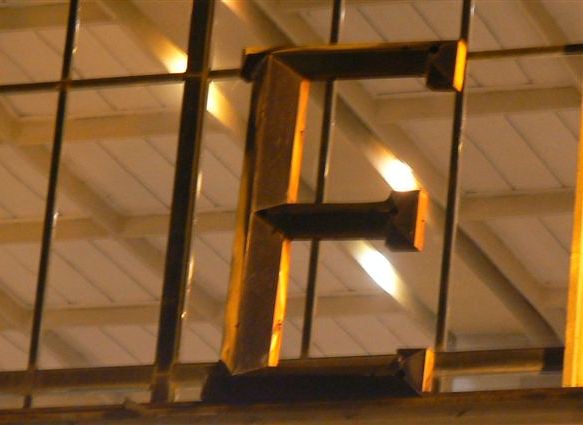The image depicts a large, freestanding, block letter "E" that appears to be metallic and painted in a golden-brown hue, catching reflections from overhead lights. The "E" is affixed along its bottom stroke. Positioned centrally in the photograph, the letter stands out against the somewhat blurry background. Behind the "E," a large window with multiple vertical and horizontal bars forms a grid, through which the interior of a building is visible. The ceiling inside showcases off-white or beige-ish tiles or panels, held up by light brown or tan beams that create a network of squares and rectangles. Blurring around the edges is noticeable, attributed to the bright illumination from three large lights affixed to the rafters, casting a glow across the scene.